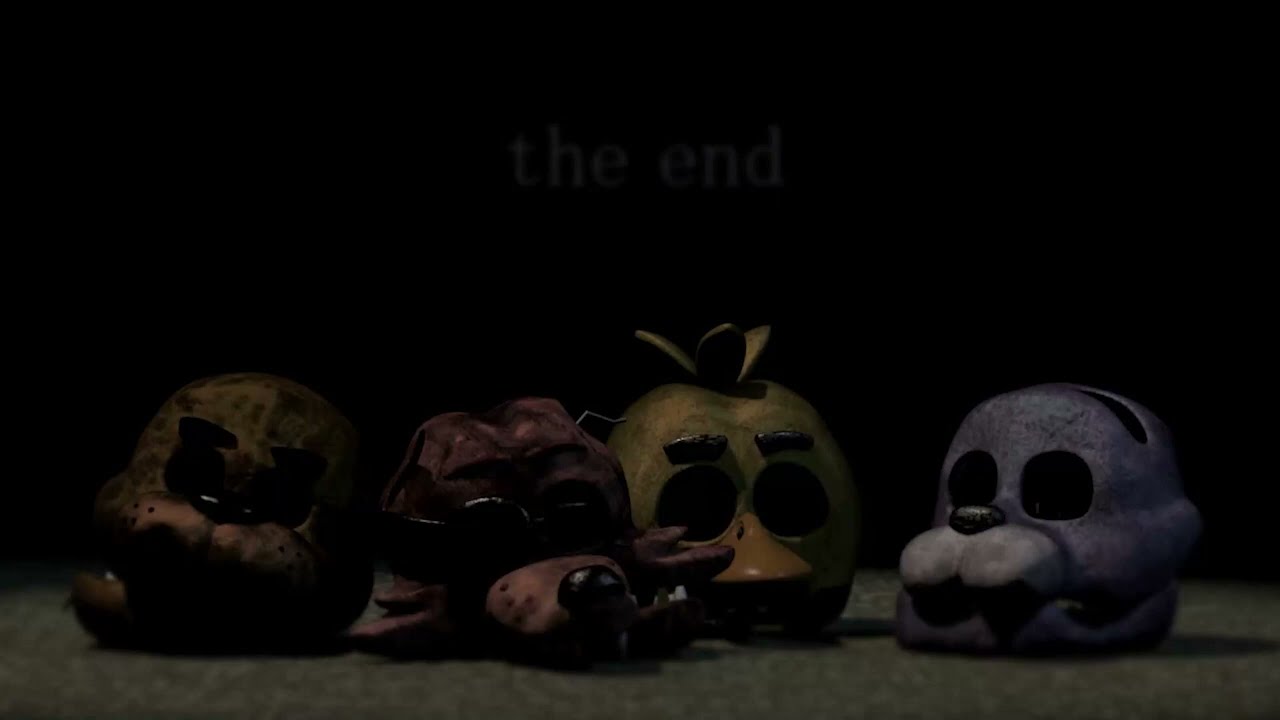In the dimly lit image, there are four ceramic animal heads arranged in a row, each resembling a hollow mask. From left to right, they are painted in various colors: green, brown, yellow, and purple. The green head appears somewhat primitive in design, while the brown one seems to depict a dog, complete with a black-painted nose and what looks like sunglasses. The yellow head resembles a duck, featuring an orange beak, black eyebrows, and three tufts of hair on top. The purple head appears to be a seal with a black nose. Each mask has large, hollow eye sockets, giving them a skull-like appearance, but they're clearly ceramic renditions rather than actual skulls. They rest on a grayish surface, with a faint, almost imperceptible "The End" text visible in white against the dark background. The overall setting is reminiscent of a scene from a horror-themed video game, akin to "Five Nights at Freddy's," adding a sense of eerie anticipation and mystery. The masks have a worn, dirty look, enhancing the unsettling atmosphere.